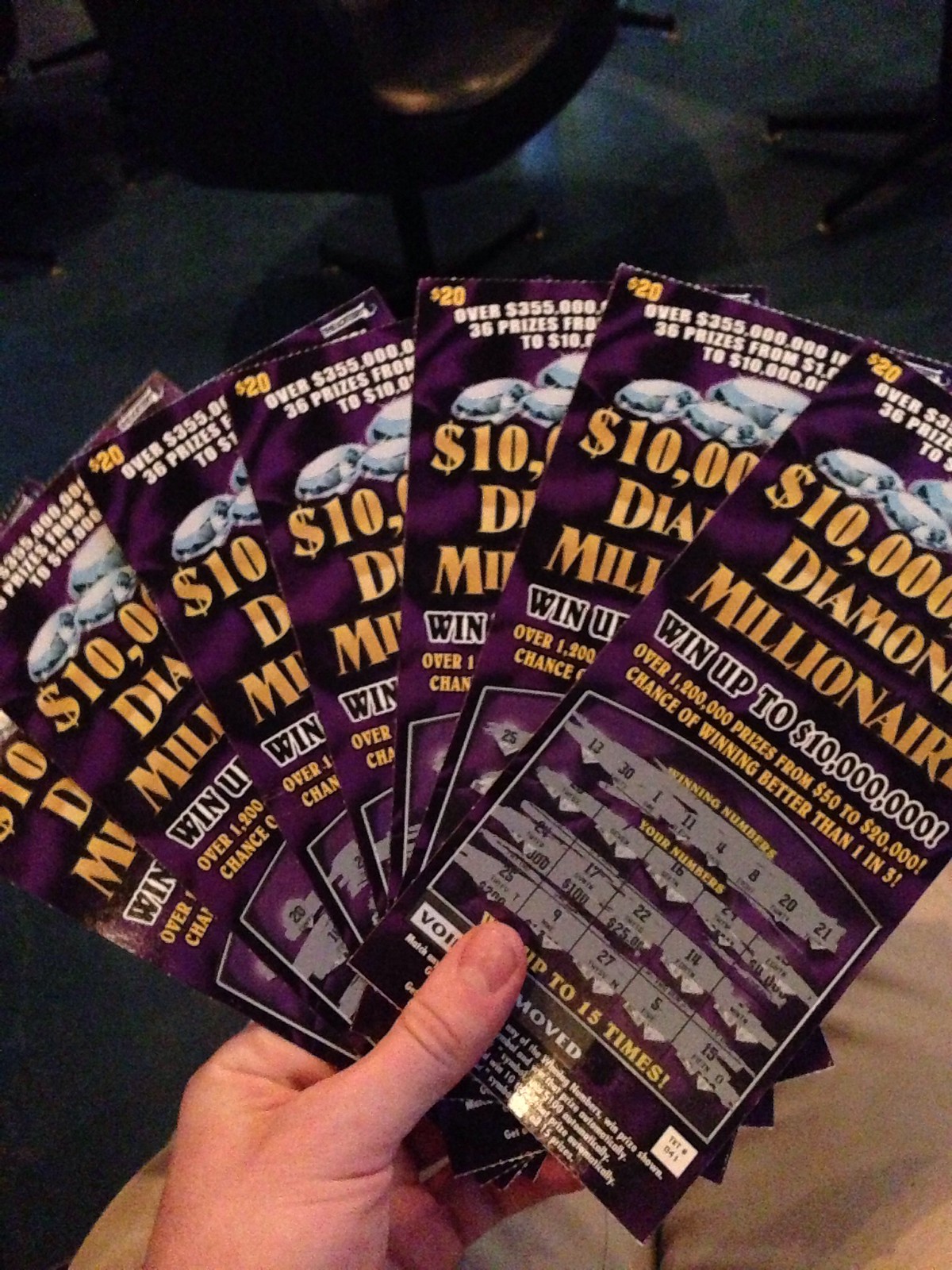The photograph captures the left hand of a white male holding a fan-like spread of seven scratch-off lottery tickets. Each ticket, emblazoned with "Diamond Millionaire" and boasting a potential prize of up to $10 million, appears to have cost $20. The tickets feature a lavish gold and purple color theme, and all have been scratched to reveal their numbers, although it is unclear if any won. The backdrop suggests the photo was taken in an office environment, indicated by the blue carpeted floor and the presence of black rolling office chairs. In the lower right corner of the image, part of the person’s light brown pants is visible, adding to the casual, indoor atmosphere.